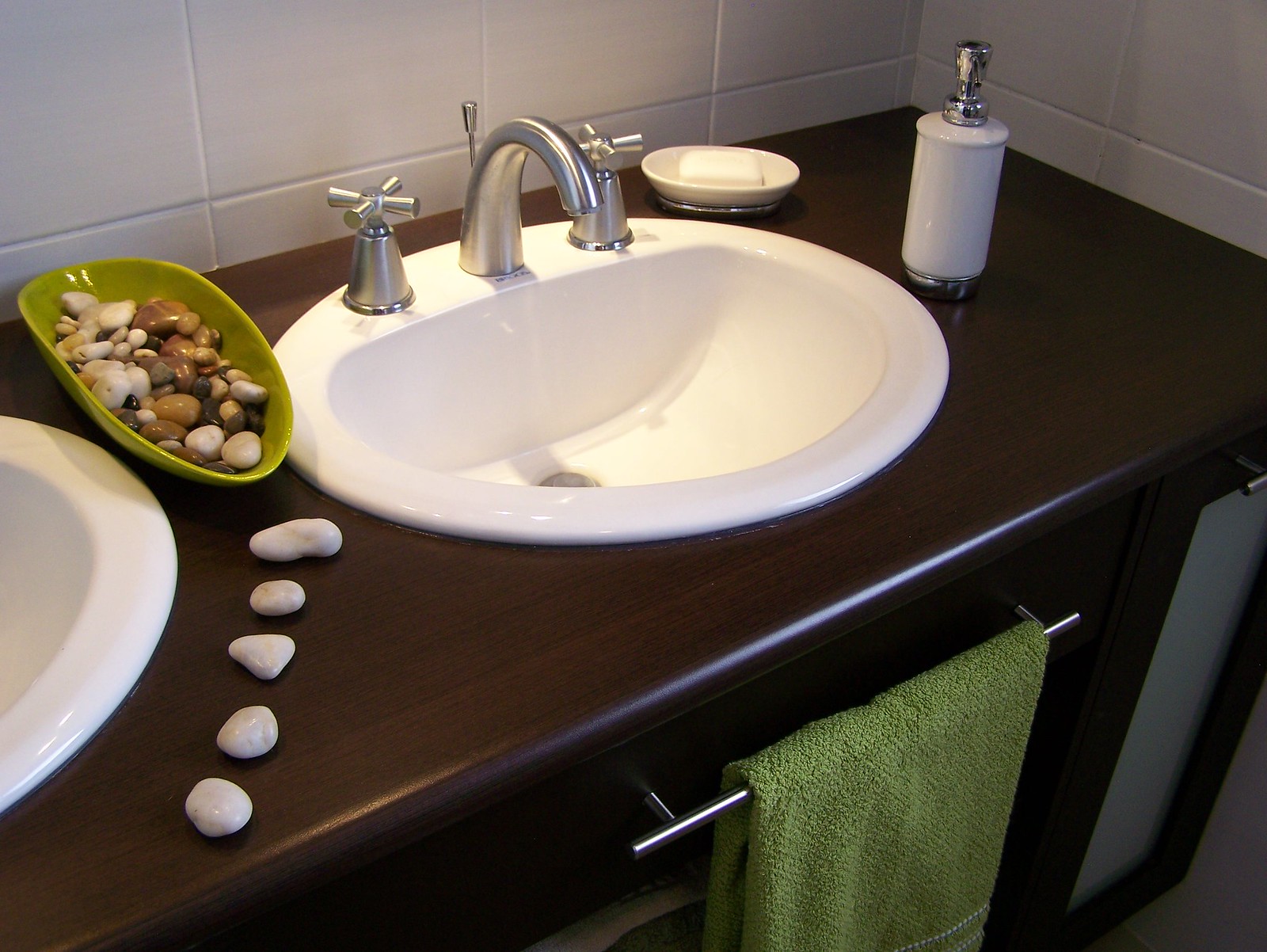The image portrays a pristine bathroom scene centered around an immaculate white ceramic sink, set against the backdrop of two intersecting gray-tiled walls, likely with 12-inch tiles. The sink is mounted on a smooth brown countertop located at the meeting point of the two walls. Prominently featured in the perfect center of the photograph is the sink, equipped with a sleek, silver metal faucet and two star-shaped knobs for controlling hot and cold water on either side.

To the right of the sink, a small dish holds a bar of soap, while just beyond it sits a squeezable soap dispenser, conveniently placed for easy access. On the left side of the sink, an oval dish contains an assortment of polished ocean agates, their smooth surfaces adding a touch of nature-inspired elegance. Five additional smooth stones artistically arranged lead the eye from the sink down to the left corner of the image.

Just visible in the top left corner is the edge of a second sink, indicating a double-sink setup in this bathroom. Below the main sink, a bar with a neatly folded green towel provides a hint of color and function. The area beneath the sink also suggests additional storage space, completing the organized and aesthetically pleasing bathroom scene.